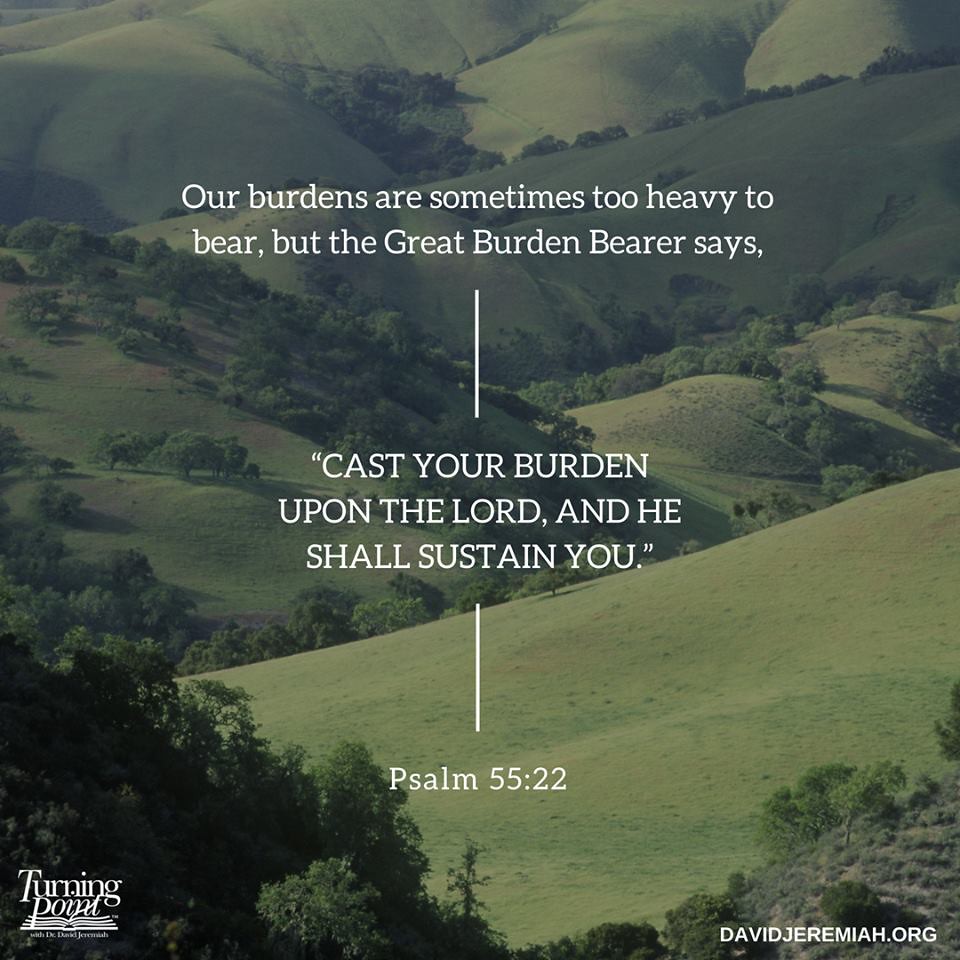This image features an inspirational and motivational spiritual quote set against a serene backdrop of rolling hills and lush, green meadows that stretch as far as the eye can see. No crops are visible, making it an ideal grazing land for sheep or cows. Centered in white text, the quote reads, "Our burdens are sometimes too heavy to bear, but the great burden bearer says, cast your burden upon the Lord and He shall sustain you," from Psalm 55:22. Below the quote, a credit notes that the image is from davidjeremiah.org. In the bottom left corner, a white logo features the name "Turning Point," depicted above an open book.